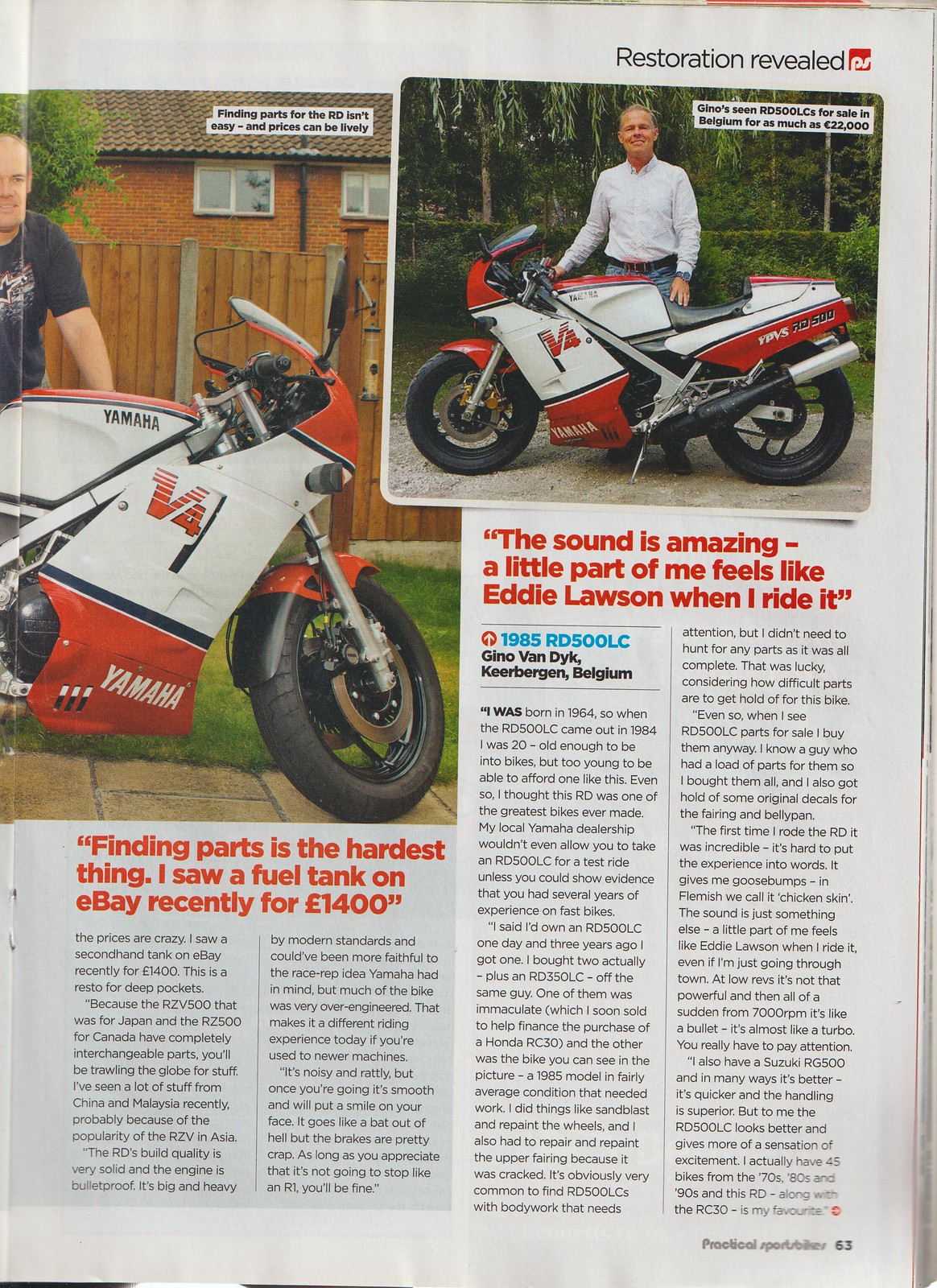This detailed magazine page features an article titled "Restoration Revealed" prominently displayed in the top right corner. The page is primarily white, and you can see staples in the crease where the left page is folded under. Two images capture the focus: the main photograph showcases an older man in a long sleeve button-down shirt and jeans, smiling as he confidently poses behind a red and white Yamaha motorcycle with "V4" emblazoned on its side. This visually striking bike is set against a backdrop of trees and hedges.

To the lower left, another photograph features the same man with the motorcycle, captioned in red, "Finding parts is the hardest thing. I saw a fuel tank on eBay recently for 1,400 pounds." An article beneath these images discusses the challenges of restoring such bikes, highlighting the spirited quest for rare parts. The text includes vivid quotes, such as "The sound is amazing. A little part of me feels like Eddie Lawson when I ride it," capturing the enthusiasm and passion of the motorbike enthusiast. Two columns of text further delve into the intricacies of the restoration process, topped with practical advice and anecdotes. At the very bottom of the page, "Practical Sports Bikes 63" is noted, linking the content to its source within the magazine.